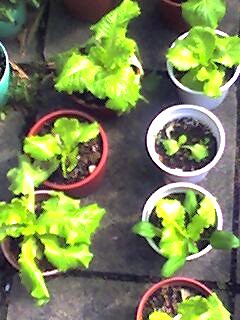This photograph, taken from a top-down perspective, showcases a collection of potted plants arranged on a slate stone patio. The image, despite being of low resolution, clearly captures a variety of red and white pots placed on square gray cement pavers. The primary focus reveals seven pots, filled with dark brown potting soil and sprouting with plants that resemble cabbage or lettuce leaves, characterized by their light to dark green coloration with white streaks. The plants exhibit varying sizes, with some having small newly sprouted leaves, while others have large leaves sprawling over their pots. On the right side of the image, a row features a terracotta pot at the bottom and three white plastic pots, which could be disposable cups, above it. To the left, there are large leafy plants partially covering terracotta pots and a white pot that appears to resemble a small vat. A bright blue pot is also visible on the left edge of the photograph, adding a splash of color to the scene. The overall arrangement highlights a mix of gardening endeavors, showcasing both budding and flourishing growths in an organized pattern.